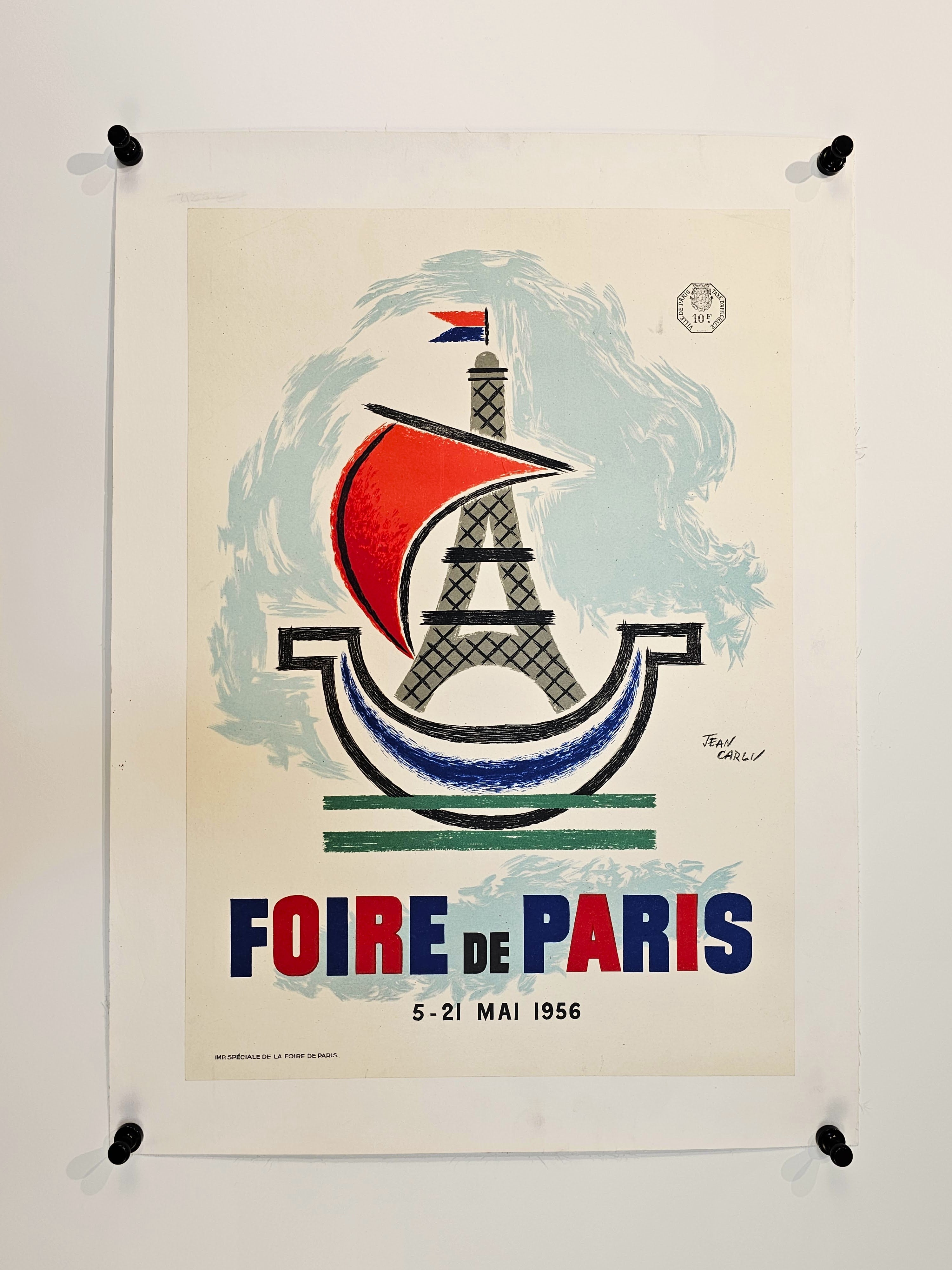This image is a photograph of an art print mounted on a white wall using four thumbtacks, one in each corner. The print itself has dimensions that could range from 8.5x10 to 11x17 inches, with a 1-1.5 inch white border framing a cream-colored background. Dominating the center of the image is an artistic depiction of the Eiffel Tower with a red sailboat-like feature and a red and blue flag at the top. Surrounding the tower are streaky, blue brushstrokes, giving an impression of sky or clouds. There is an additional detail in the top right corner that appears to be hand-stamped, but it's too small to decipher clearly. Alongside the Eiffel Tower, the phrase "FIOR DI PARIS" is prominently displayed in alternating red and blue letters, with the date "5-21 MAI 1956" written in smaller letters beneath it. The artist's signature, "JEAN CARLEY," can be found to the right of the image. There's also a line of text in the bottom left corner that is too small to read. The main colors in the print are white, black, red, and blue, creating a striking visual composition likely intended as an advertisement or art piece.